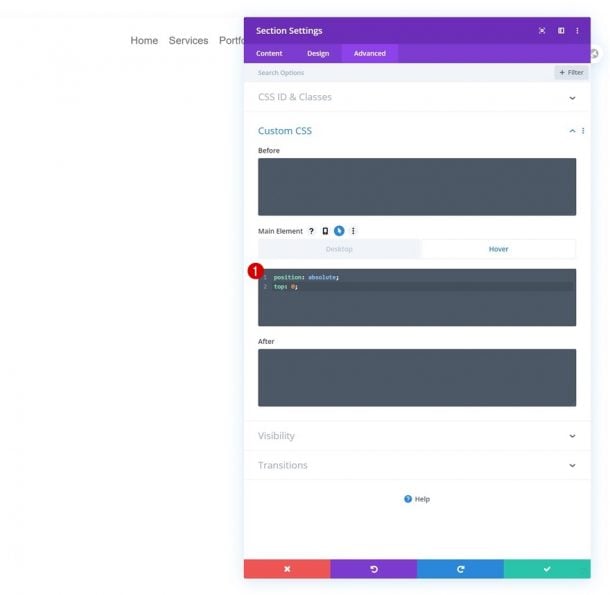The image depicts a user interface with various settings and options in a stylish, modern design. On the right side, there's a pop-up window featuring a dark purple header labeled "Section Settings" in white text. Adjacent to this label, on the right, there's a white "X" symbol within a bolded area for closing the pop-up. Following this is a partially filled square icon with an apparent blank space on the right, and next to it, three vertical dots symbolizing a drop-down menu.

Below the main header is a smaller, lighter purple sub-header. This area contains three white menu options: "Content," "Design," and "Advanced." The "Advanced" option is highlighted in an even paler purple, indicating it is currently selected. Underneath, a light gray banner reads "Search Options" on the left, with a filter option on the right.

Further down, a white strip displays the text "CSS ID & Classes" in light gray capital letters, followed by a down-pointing black arrowhead indicating a drop-down menu. Below this, on the left, the label "Custom CSS" appears in a navy blue font. Adjacent to it is the word "Before" in small, bold black letters, followed by a large dark gray rectangular input area.

Directly beneath the rectangular area, the text "Main Element" appears in bold black lettering, next to a light gray background icon featuring a question mark. Beside the question mark icon is another icon resembling a mobile device, followed by a blue circle containing a cursor icon. Finally, on the far right, there are three vertical dots signifying another drop-down menu.